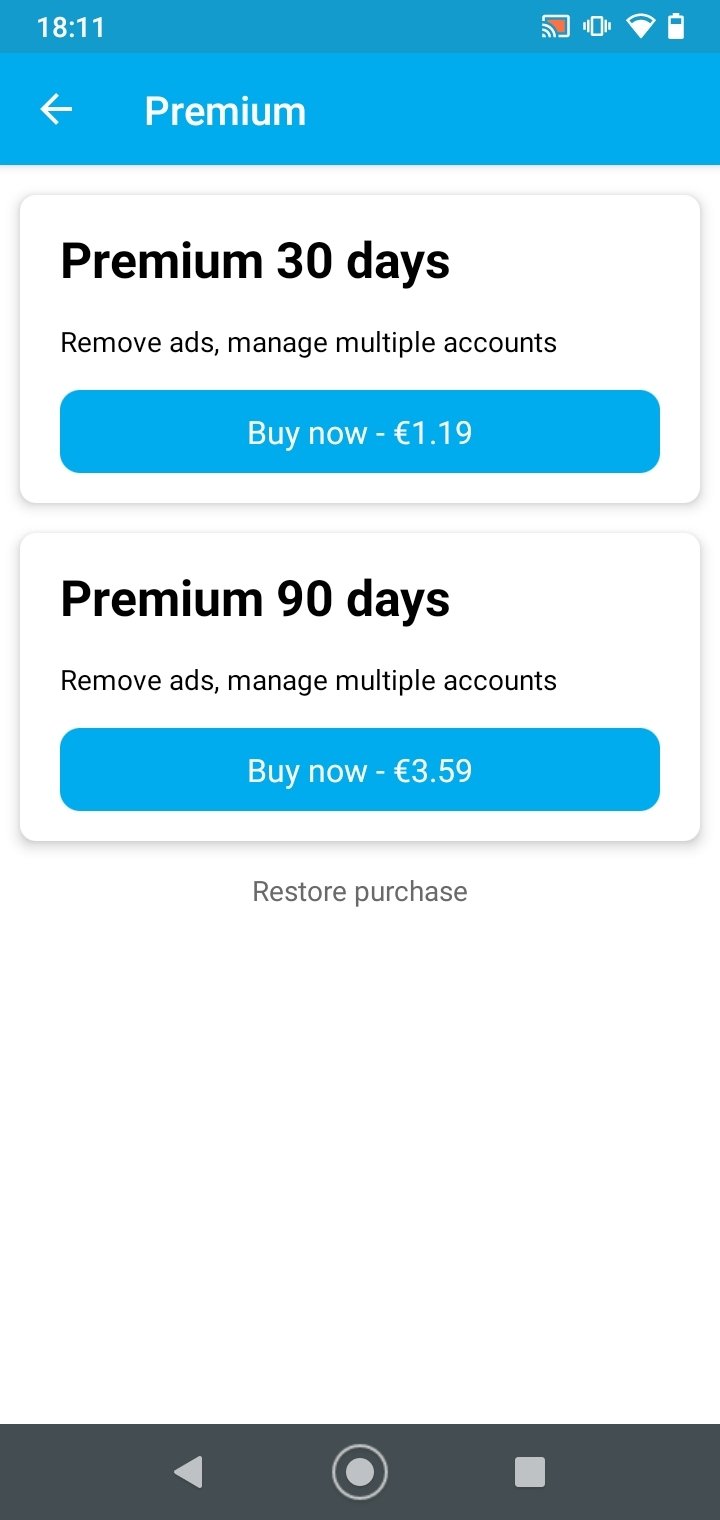In the image, the top portion features a blue header with the word "Premium" written in white on the top left. Adjacent to this is a white back button. Below the header, the main content area of the page has a white background and is divided into two sections offering subscription options.

The first option is centrally located just below the blue header. It is a premium package for 30 days, written in black text that reads, "Premium 30 days - Remove ads, manage multiple accounts." Below this, in a blue button, it says "Buy Now - 1.19 euros."

The second option, positioned below the first, offers a premium package for 90 days. The text in black reads, "Premium 90 days - Remove ads, manage multiple accounts," followed by a blue button stating "Buy Now - 3.59 euros."

At the bottom of the page, there is an option written in black text that reads "Restore Purchase." The overall background of the image is white except for the blue header, and the page layout appears to be from a smartphone interface.